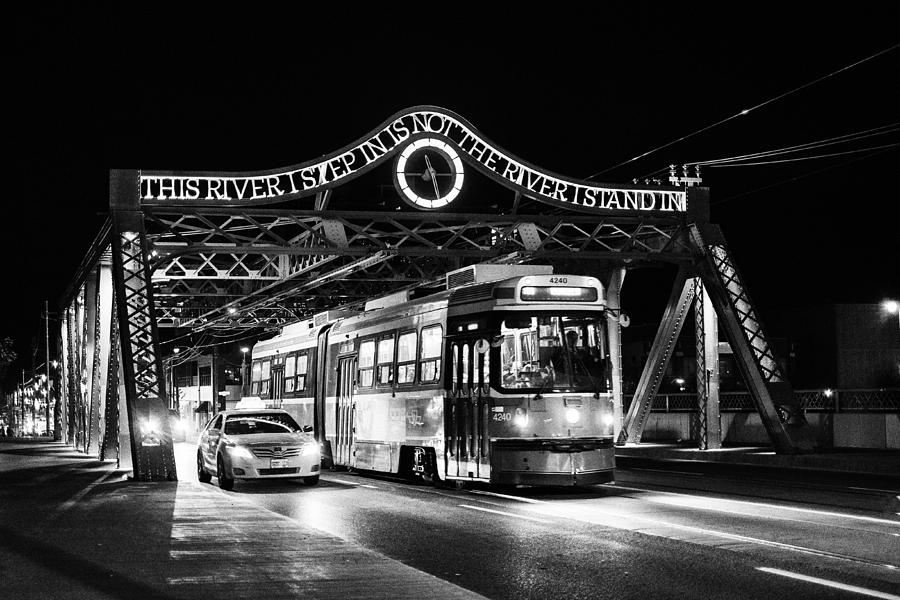In this black-and-white nighttime photograph, two vehicles—a car and a bus—are captured driving side by side across a short, two-lane bridge with a steel lattice design. The entire scene is enveloped in pitch darkness, except for distinct illuminated features. The bridge spans a river, and an illuminated sign overhead reads, "This river I step in is not the river I stand in." Below the sign, a clock with a glowing rim is also visible, although its numbers are obscured by the darkness. Both vehicles have their headlights on, and additional light from behind suggests the presence of more cars. The bridge, not very high and possibly resembling a one-way bridge due to the darkness concealing any opposing lanes, has parts of its structure lit, adding to the atmospheric feel of the image.